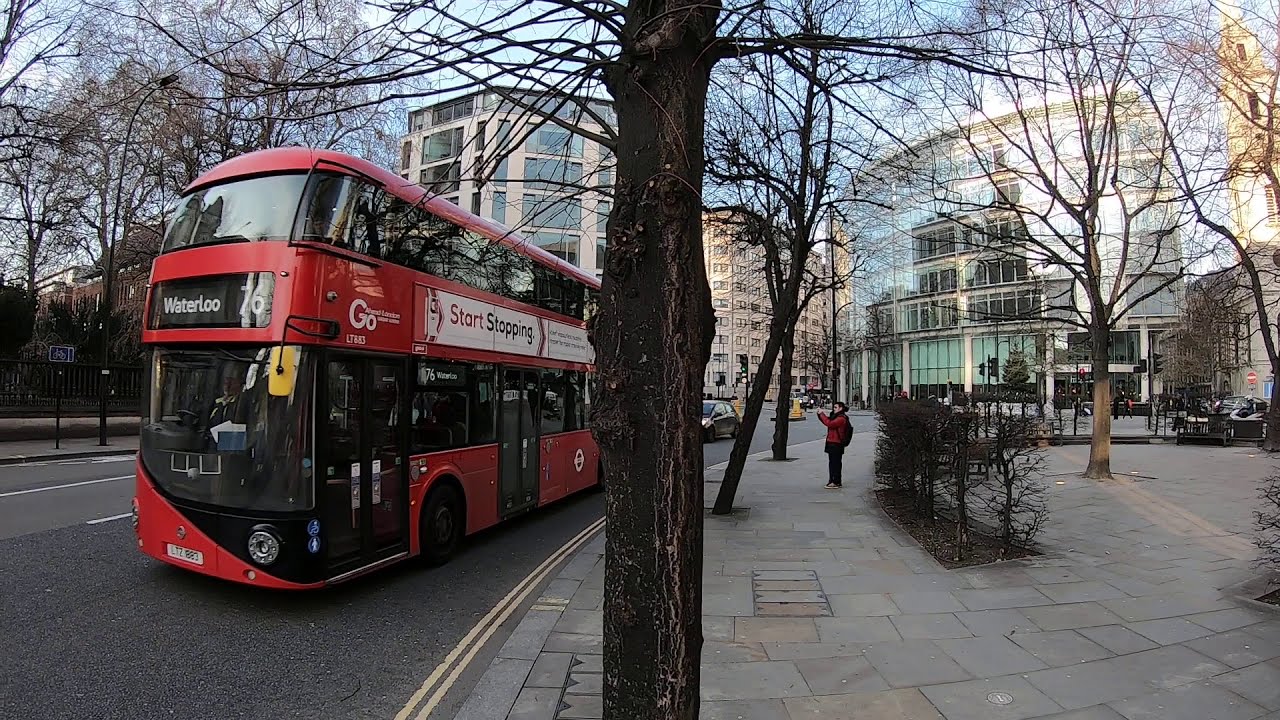In the image, a red double-decker bus marked "76 - Waterloo" is driving along the left side of a bustling street. An advertisement on the bus's side encourages onlookers to "start shopping." The street is flanked by a spacious cement or tiled sidewalk. A tree trunk emerges from the center of the sidewalk, which stretches to the right side, where leafless trees stand. A woman wearing a red coat and black pants is captured in mid-action, seemingly photographing the bus. The background features several tall, white buildings with numerous glass windows, under a partly cloudy blue sky. The scene suggests a bright, sunny, and somewhat chilly day in the city.